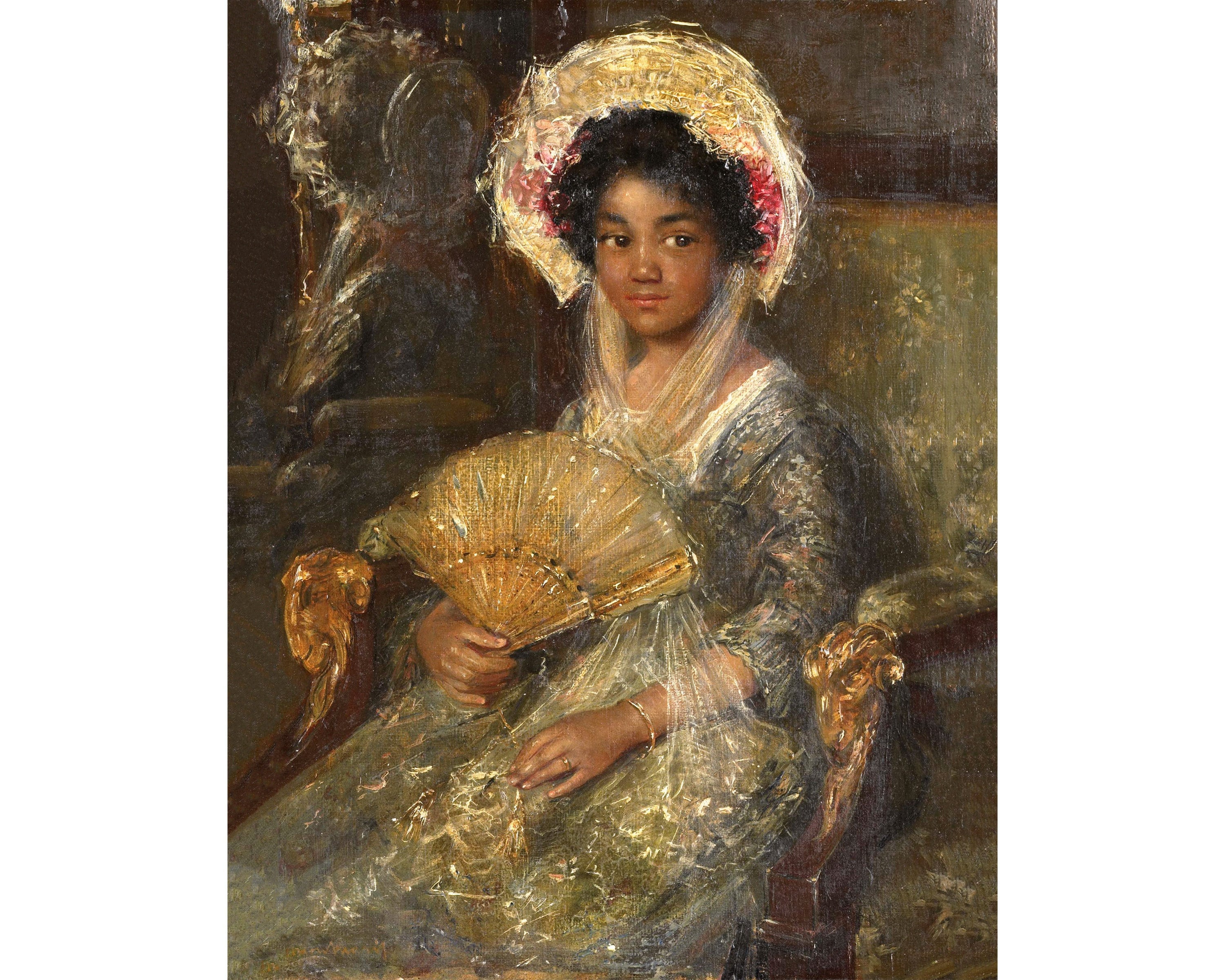This detailed portrait illustrates a young African-American girl from the Victorian era, gracefully seated in a regal, upholstered chair with gold embellishments and wooden arms. The chair, which features nailhead upholstery, is a muted olive green color, complementing the detailed gown she is wearing that appears to be an olive green or a silvery-gold hue. The girl has dark, curly hair adorned with a wide-brimmed sun hat embellished with flowers and a see-through taffeta veil. Her dark brown eyes gaze inquisitively to the side, not directly at the viewer, hinting at her contemplative mood. She accessorizes with a bracelet on her wrist and a ring on her finger while delicately holding a golden hand fan. The background is dark and somewhat blurred, possibly featuring a stone statue or carving, adding depth and historical context to the scene. There is a mirror behind her, reflecting her image and enhancing the portrait's ornate and elegant ambiance.